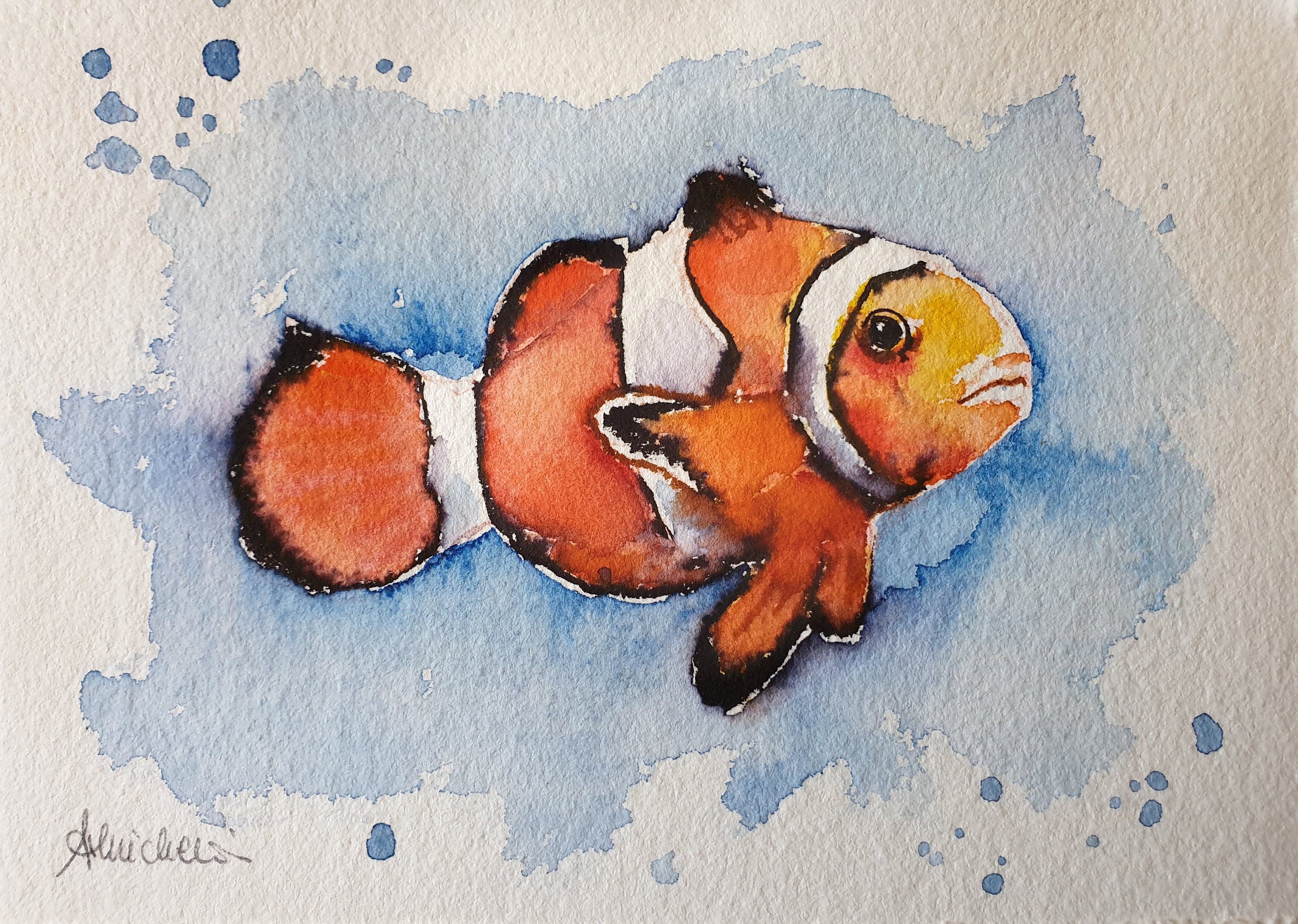This image depicts a landscape-oriented watercolor painting on a textured, porous paper background that is a light gray or white color. At the center of the painting is a detailed rendition of a clownfish, which has been described by some as a goldfish, but is accurately a clownfish, characterized by its distinct orange and white stripes. The fish faces right, and its body features three wide white stripes that contrast against the vibrant orange. Black detailing outlines the tip of the tail, dorsal fin, and lower fins. Its eye, looking directly at the viewer, is black, while its mouth appears silvery. The background surrounding the fish consists of splotches of watery blue watercolor, giving the impression of the fish swimming. This blue appears lightly splashed or spilled, with some edges still showing the untouched white paper. In the bottom left-hand corner, the artist’s signature is present, written in cursive and difficult to read, but looks like "A-L-I-U" for the first name and "C-H-E-T" something for the last name.